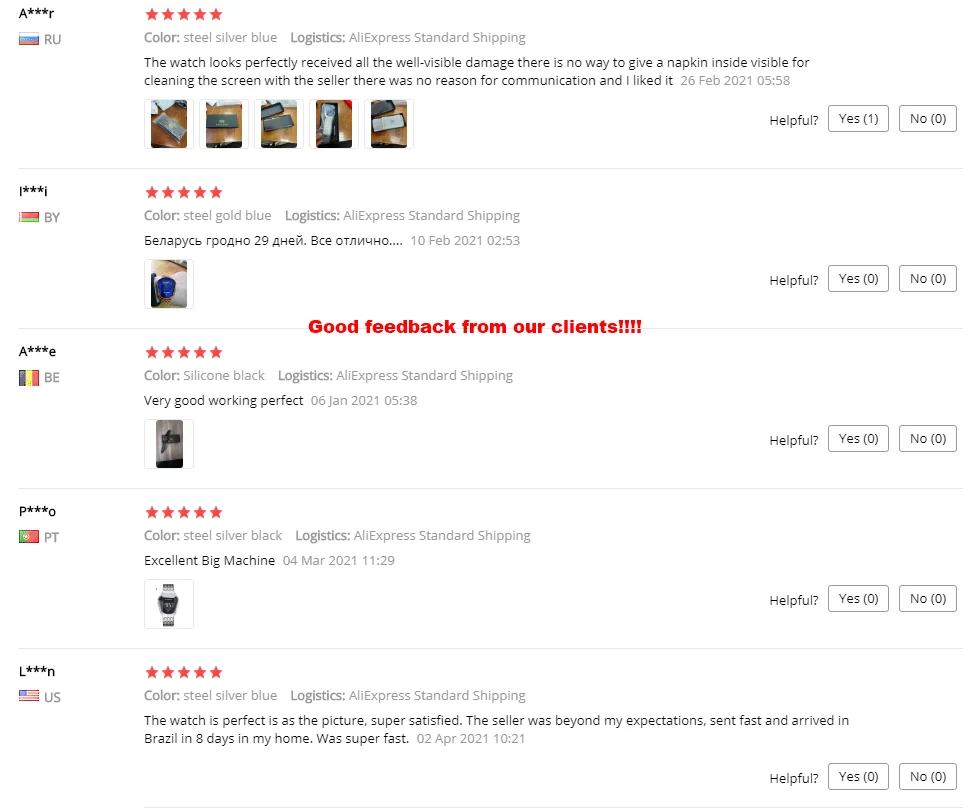The image displays five client feedback entries for a product, presumably a watch, on a white background. Some of the reviews are partially in Russian. Each review is rated five stars, as indicated in red above each response.

1. **Review 1**: The first review features text in Russian and mentions details such as "RU," "color: steel, silver, blue," "logistics: AliExpress standard shipping." Despite some visible damage, the product (a watch) was received in good condition. The reviewer noted the absence of a cleaning cloth within the package. The interaction with the seller was deemed unnecessary. This feedback is dated February 26, 2021, at 5:58. Accompanying images show the watch in its box before and after unboxing, placed on a brown table. One person marked this review as helpful.

2. **Review 2**: The second review mentions "color: steel, gold, blue" and follows with text in Russian which remains untranslated. The logistics are again noted as AliExpress standard shipping. This review is dated February 10, 2021, at 2:53. It did not receive any helpfulness marks.

3. **Review 3**: Located under the header "Good feedback from our clients," highlighted in red with four exclamation marks. This review mentions "color: silicone, black" and "logistics: AliExpress standard shipping." The review simply states, "Very good, working perfect," dated January 6, 2021, at 5:38, with no helpfulness marks.

4. **Review 4**: This feedback mentions "color: steel, silver, black" with the logistics again being AliExpress standard shipping. It reads, "Excellent big machine," dated March 2021 at 11:29, without marks for helpfulness.

5. **Review 5**: The final review highlights "color: steel, silver, blue" with AliExpress standard shipping logistics. The reviewer expresses high satisfaction, stating the watch matched the description and exceeded expectations. They praise the fast delivery, which took only eight days to reach Brazil. This review is dated April 2, 2021, at 10:21, without helpfulness marks.

Each review praises the product, with emphasis on its appearance and functionality, reinforcing the overall positive reception from the clients.